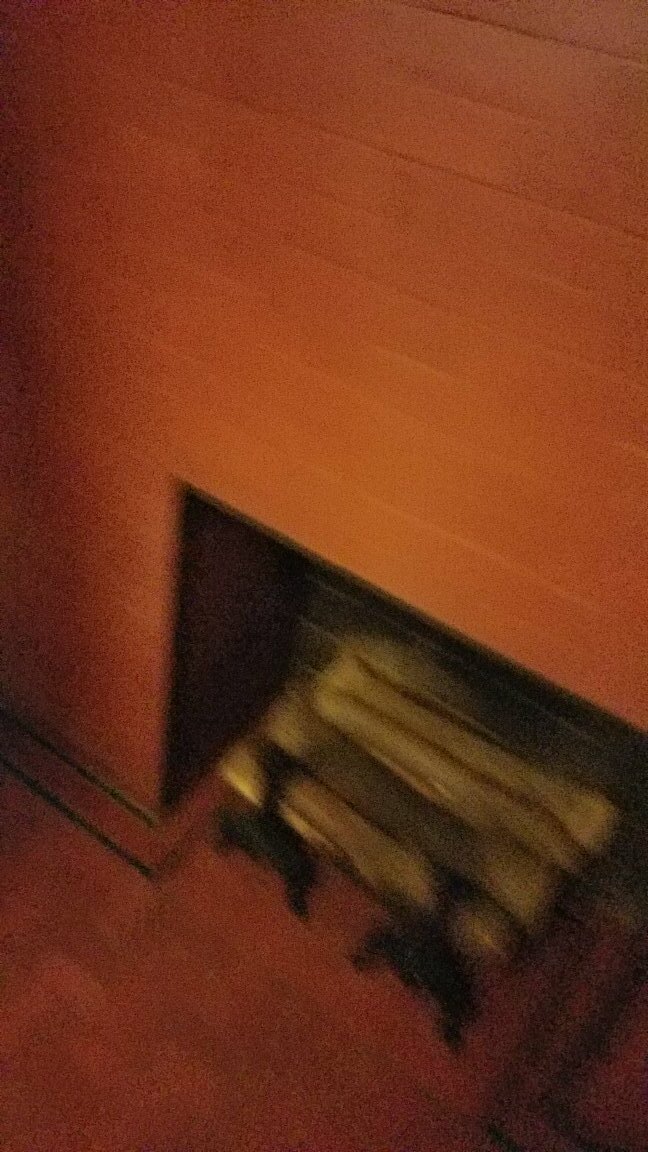This photograph captures a blurred interior setting, likely showcasing a fireplace. The indistinct quality of the image makes it difficult to discern precise details, but a darker section is visible, possibly representing the fireplace opening set against a vibrant red or orange wall. The overall composition suggests the picture was taken hastily or in low light, contributing to its lack of clarity. Within the obscured dark area, there appear to be objects that might be logs or fireplace tools. The warm color palette evokes a cozy atmosphere, while the blurred elements impart a sense of mystery and intrigue.